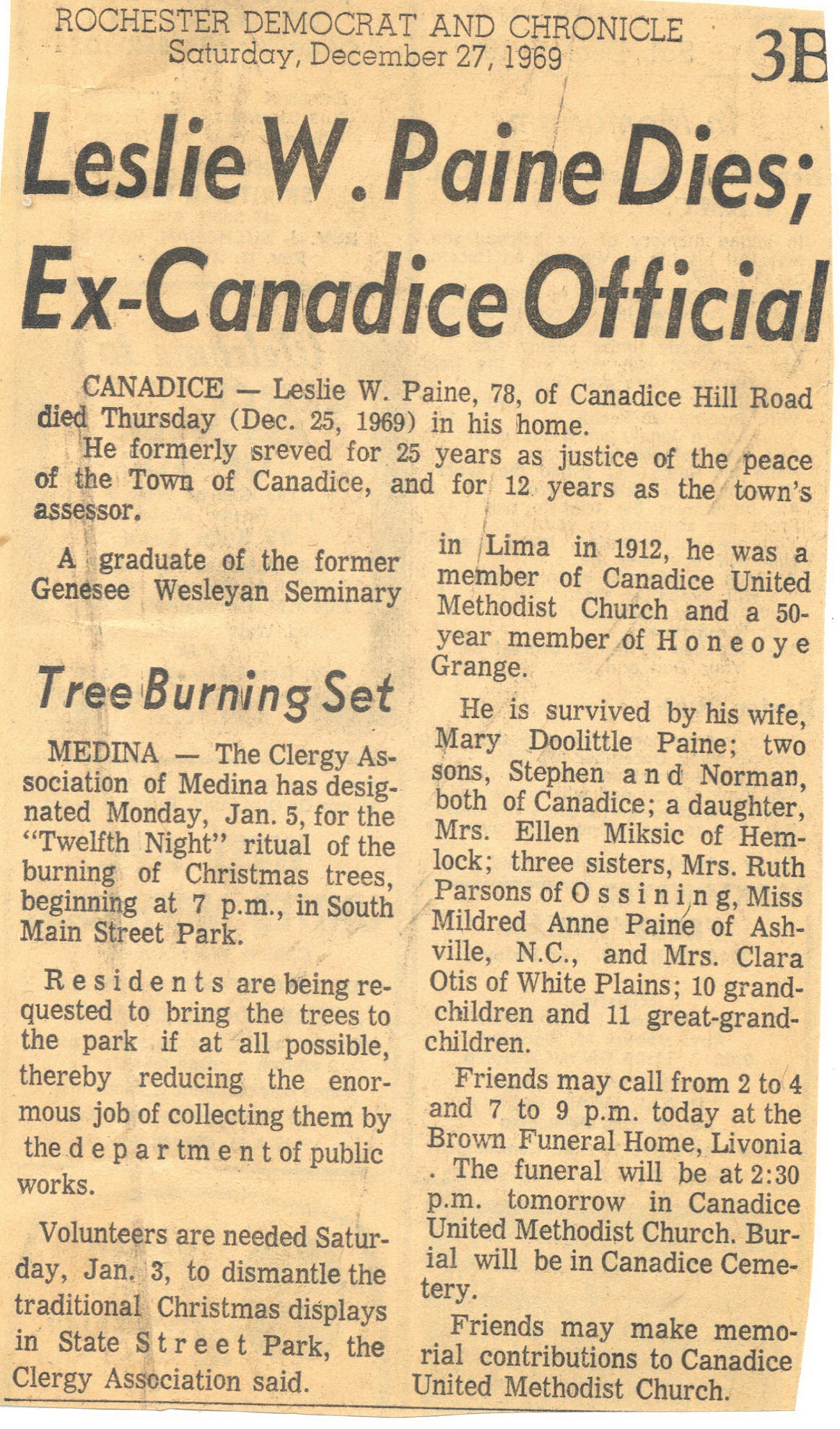The image is a rectangular scan of a faded newspaper clipping from the Rochester Democrat and Chronicle, Saturday, December 27, 1969, with a prominent "3B" on the right side of the header. The headline reads "Leslie W. Payne Dies, Ex-Canadice Official." The article details the obituary of Leslie W. Payne, 78, of Canadice Hill Road, who passed away at his home on Thursday, December 25, 1969. Payne served for 25 years as Justice of the Peace in Canadice and for 12 years as the town's assessor. A 1912 graduate of the former Genesee Wesleyan Seminary in Lima, he was a member of the Canadice United Methodist Church and a 50-year member of the Honeoye Grange. He is survived by his wife, Mary Doolittle Payne, two sons, Stephen and Norman, both of Canadice, and a daughter, Mrs. Ellen Mixick of Hemlock, along with three sisters, Mrs. Ruth Parsons of Ossining, Miss Mildred Ann Payne of Asheville, North Carolina, and Mrs. Clara Otis of White Plains. The obituary also lists his 10 grandchildren and 11 great-grandchildren. Visitation hours were stated as 2-4 p.m. and 7-9 p.m. that day at the Brown Funeral Home, Livonia, with the funeral at 2:30 p.m. the next day at Canadice United Methodist Church and burial at Canadice Cemetery. Memorial contributions could be made to the Canadice United Methodist Church. The article concludes in the right-hand column with details about a local tree-burning event scheduled for January 5th, organized by the Clergy Association of Medina to be held in South Main Street Park.